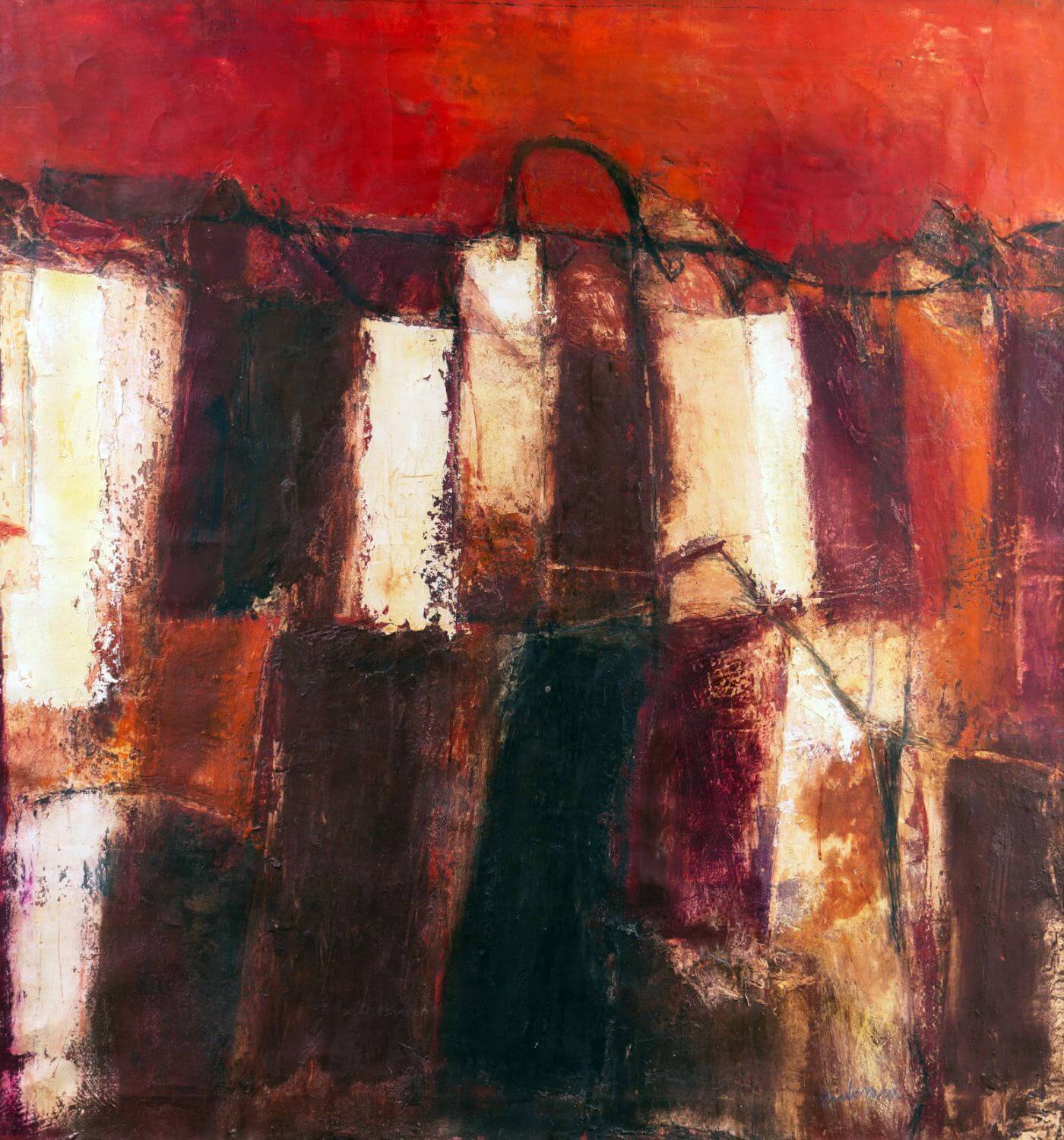This image is a rectangular Impressionist-style painting, approximately six inches tall and five inches wide, set against an orangey-red background that lightens towards the upper right corner. The central focus of the painting features a large, wide bag with a small handle sticking upward in the middle, though the painting is abstract with no clear depiction of any specific object. The bag area displays an assortment of vertical rectangles in shades of white, brown, and orange, blending seamlessly together with no distinct lines separating them. These rectangles vary slightly in width and scatter at different heights, giving a sense of randomness and fluidity. The colors within the rectangles are mixed with other tones, including deep reddish-black, cream, and a dark, burnt-looking orange, contributing to the impressionistic blending.